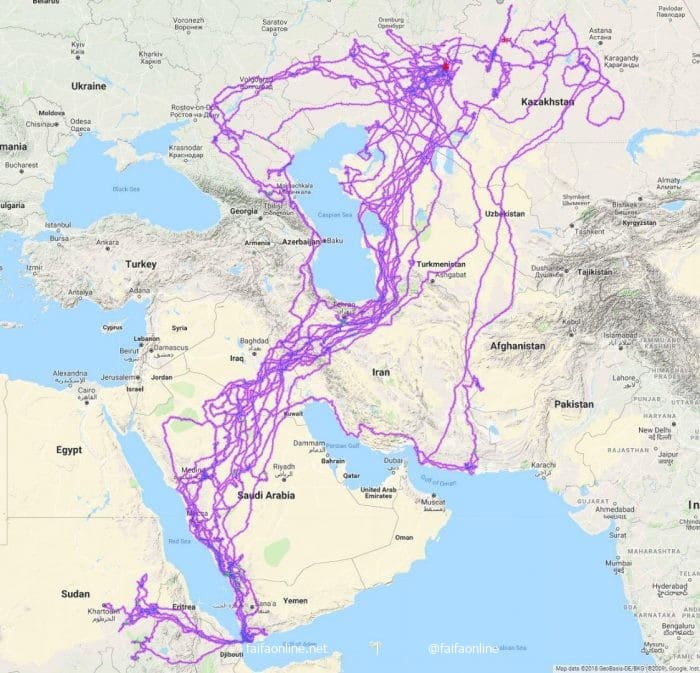This detailed map of Western Asia and parts of Eastern Europe and North Africa showcases notable countries such as Saudi Arabia, Egypt, Sudan, Iran, Afghanistan, Pakistan, Ukraine, Turkey, Syria, Jordan, and parts of India. Additionally, it includes regions such as Kazakhstan, Turkmenistan, Uzbekistan, and other central Asian countries. The map depicts topographical elements like mountain ranges and bodies of water, including the Persian Gulf, marked in blue. Overlaying the terrain are numerous purple lines, resembling tangled yarn or spaghetti, which snake around countries but avoid crossing bodies of water. These lines, possibly representing pipelines, electrical grids, or roadways, start from two red dots and expand in a web-like feature across the map. This intricate network covers the coastlines and stretches through the mainland, yet the absence of a legend renders their exact purpose ambiguous.